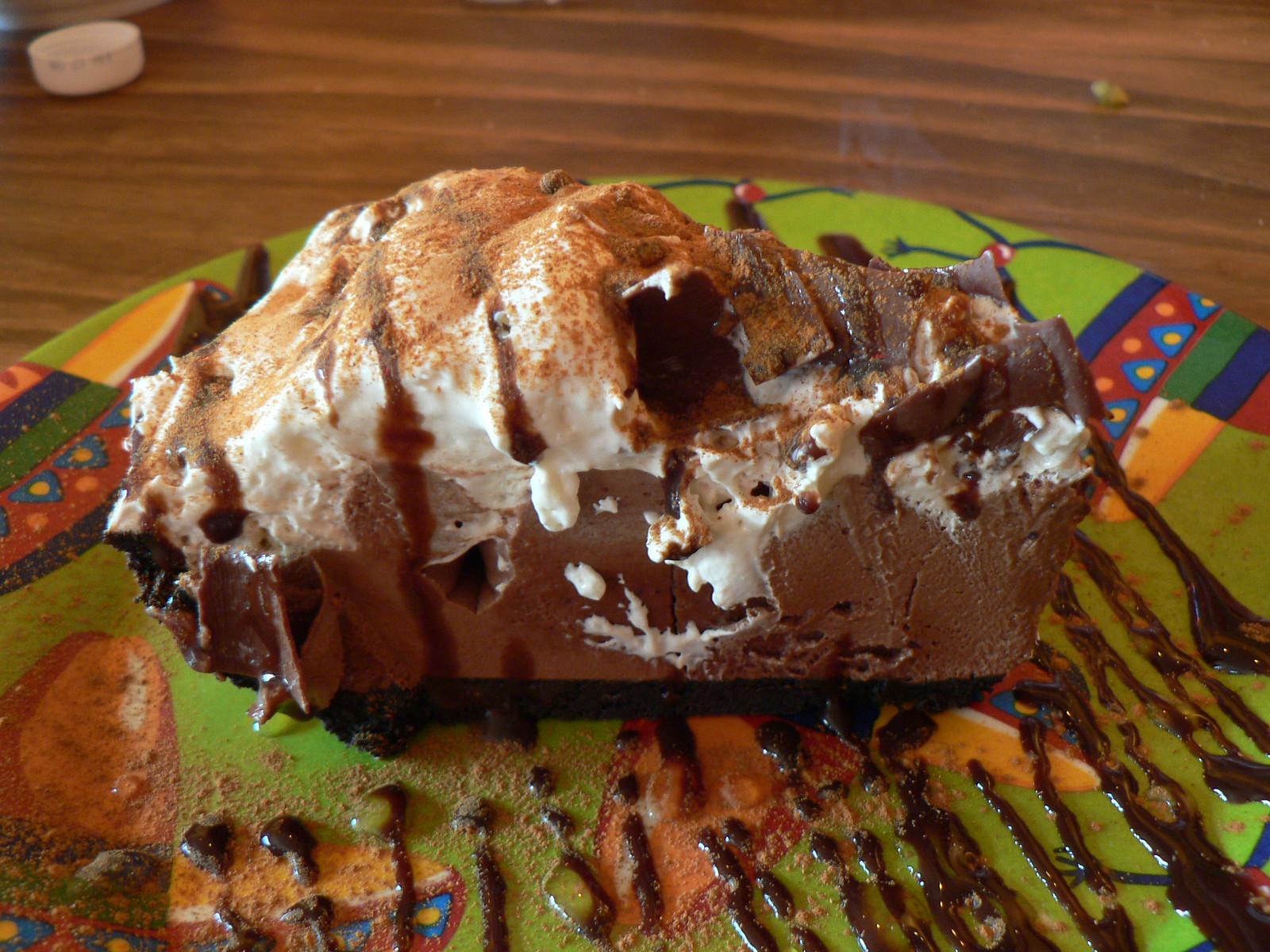The image shows a vibrant scene set on a wooden table. At the center of the picture rests a colorful, fiesta-style plate decorated with blue triangles, white dots, red areas with peach dots, yellow, green, and orange sections. On the plate is a slice of chocolate cake, adorned with white frosting and a sprinkle of cinnamon on top, suggesting an ice cream cake. Beneath and around the cake, hot fudge has been artfully drizzled, though not in a perfectly symmetrical pattern, indicating a homemade touch. In the upper left corner of the image, a white bottle cap can be seen. The setting appears to be indoors, likely in a kitchen or at a restaurant, well-lit to showcase the details of the cake and plate.